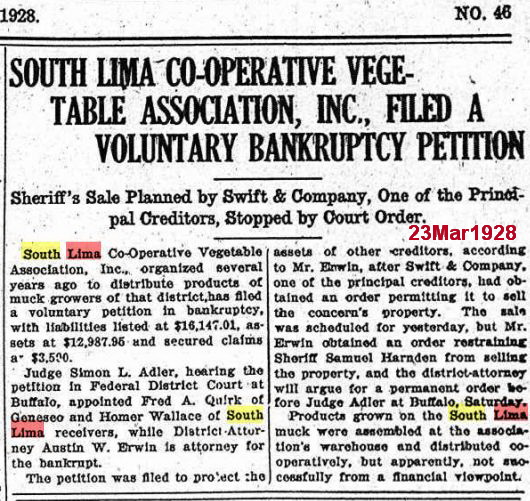This image is a digitized clipping of an old newspaper article from 1928, labeled as article number 46. The headline reads, "South Lima Co-operative Vegetable Association Inc. Filed a Voluntary Bankruptcy Petition." The subtitle elaborates, "Sheriff Sales Plan by Swift & Company, One of the Principal Creditors, Stopped by Court Order." The article is split into two sections, and the first paragraph states that the South Lima Co-operative Vegetable Association, organized several years ago to distribute products of muck growers in that district, has filed for bankruptcy. It lists the liabilities at $16,147.01 and assets at $12,987.95, with secured claims of $3,500. The article mentions the association's activities in upstate New York, specifically Buffalo, where the suit was filed and receivers were appointed. Some text in the digitized version is highlighted, suggesting the use of software for word detection.